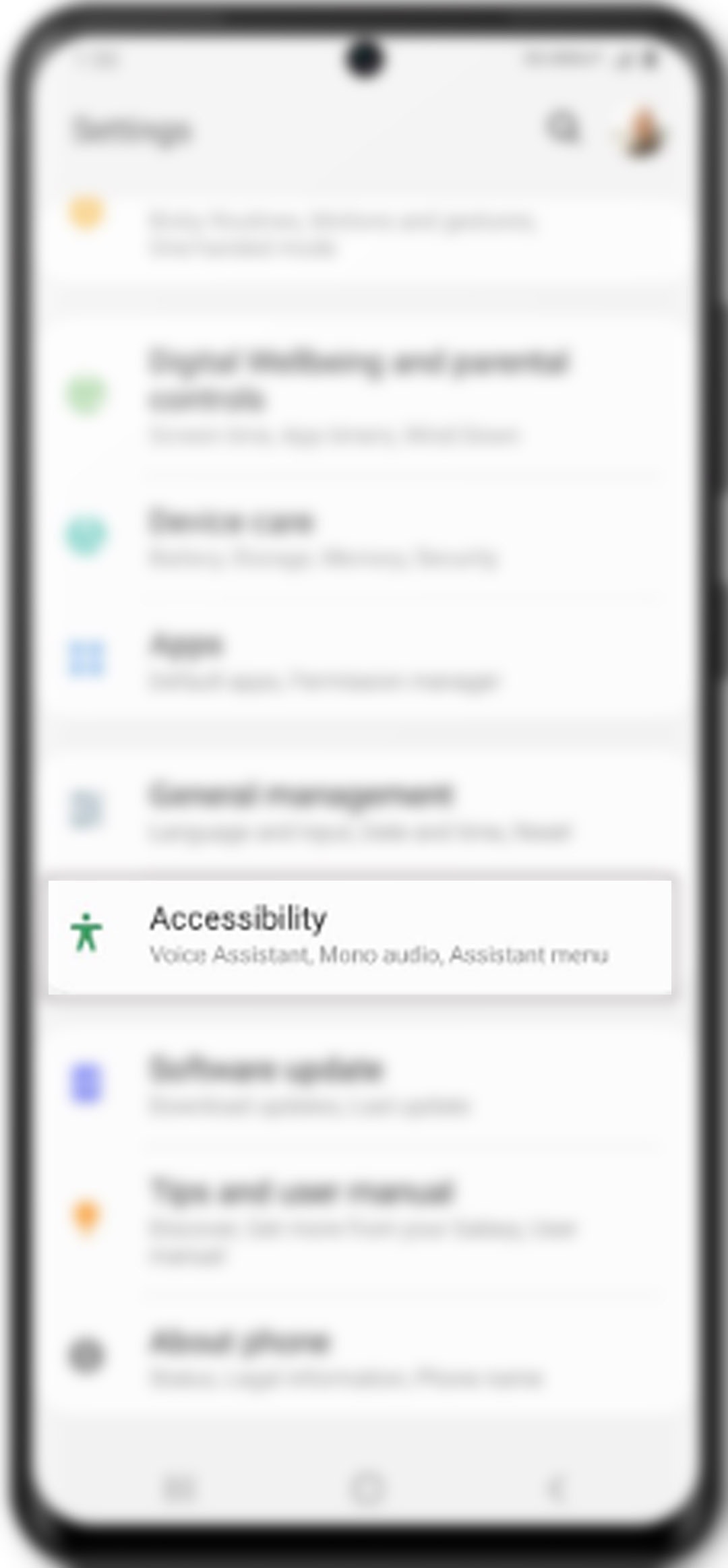The image is a vertical rectangle resembling a blurry screenshot of a cell phone's settings menu. Encased in a black border, the phone appears to be in settings mode. At the top, below the border on the right, there's a black circle indicating the account currently logged in. Most of the screen content is indistinct, except for a prominently visible white pop-up box. This box displays a green icon on the left and contains clearly legible text listing "Accessibility," "Voice Assistant," "Mono Audio," and "Assistant Menu." The remaining settings on the screen are grayed out and less readable, accompanied by small icons to their left. At the very bottom, a grayish border houses three symbols, typically indicative of common navigation buttons on a smartphone.